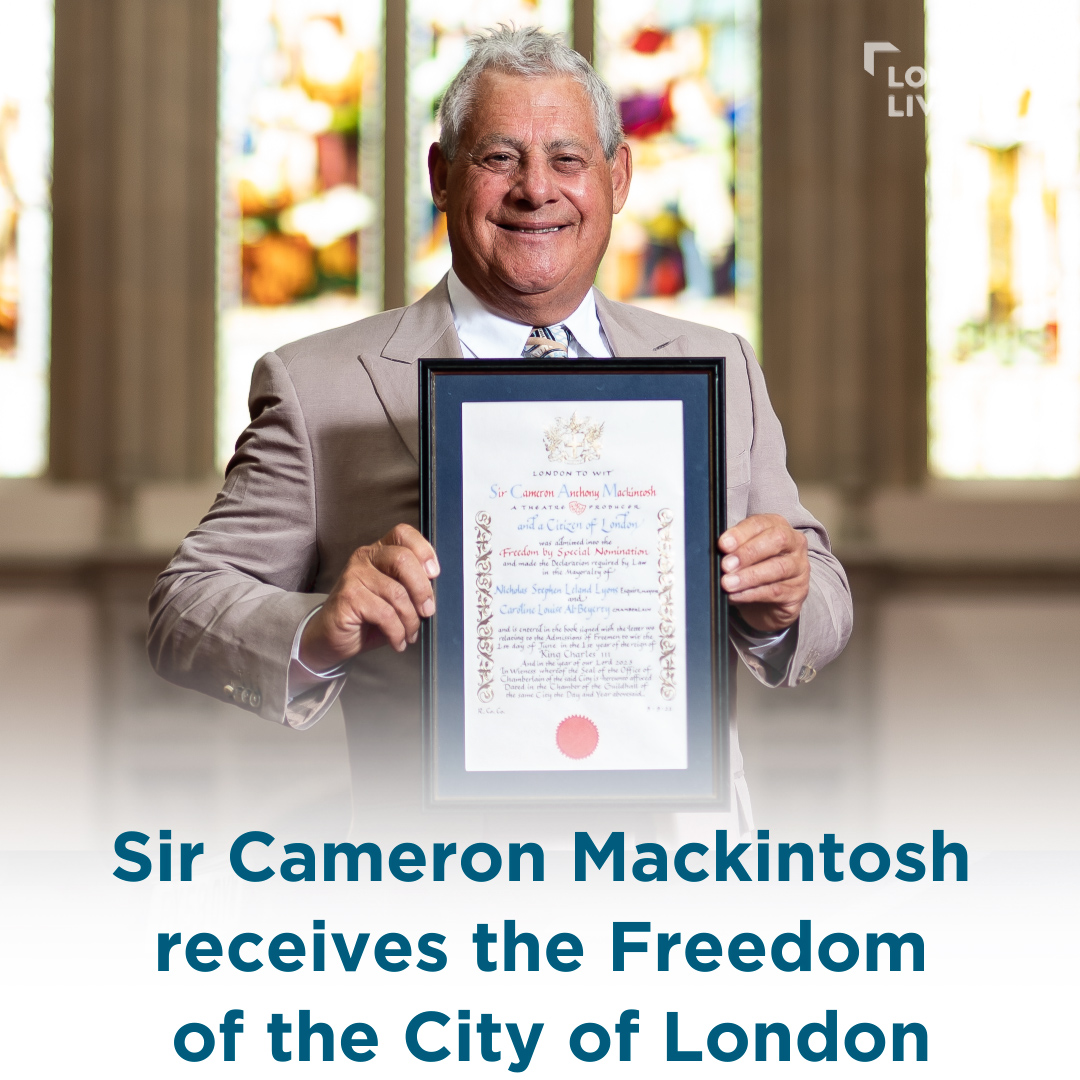In this color photograph, an elderly man, appearing to be in his late 50s to early 60s, stands smiling broadly at the camera. He has short, silver hair and wears a gray suit jacket over a white collared shirt with a visible necktie. The man is holding a rectangular framed certificate delicately by its black edges with his fingertips. The certificate text prominently features "Sir Cameron Macintosh receives the Freedom of the City of London." The background shows out-of-focus stained glass windows, adding a colorful and distinguished backdrop to the scene. A subtle watermark is present at the top right of the image, though its content is indistinct. The man's face is characterized by numerous wrinkles, highlighting his advanced age, and he appears joyful and proud, celebrating his noteworthy achievement.